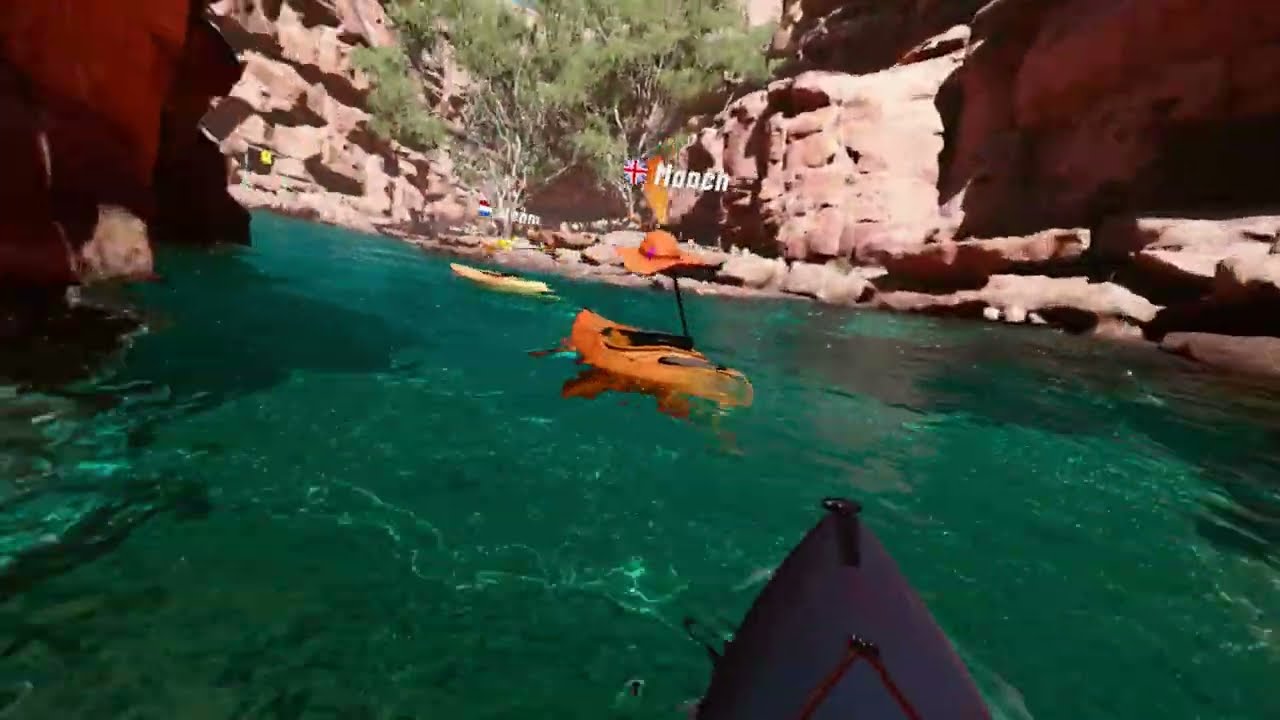This image depicts a photorealistic yet potentially animated scene of a canyon river with low resolution adding to the unclear distinction between reality and animation. The vivid, greenish-blue water flows from the bottom right to the top left of the image and is lined by towering, red-brown rock formations bathed in sunlight. Green-leaved trees are seen sprouting at the top center of the rock formations.

The viewer appears to be on a dark purple kayak, visible near the bottom right corner. Central to the image, an orange kayak faces away, seemingly paddled despite being passenger-less, and sports an orange sun hat perched where a kayaker would sit. Above the paddle, a white word and a flag overlay the scene. Ahead of this is a yellow kayak, similarly devoid of an occupant but equipped with a yellow and black paddle, also featuring white text and a flag overlay. The canyon and its trees bask in sunlight, and while the image hints at motion, the overall blurriness adds a surreal quality to the tranquil yet animated river scene.